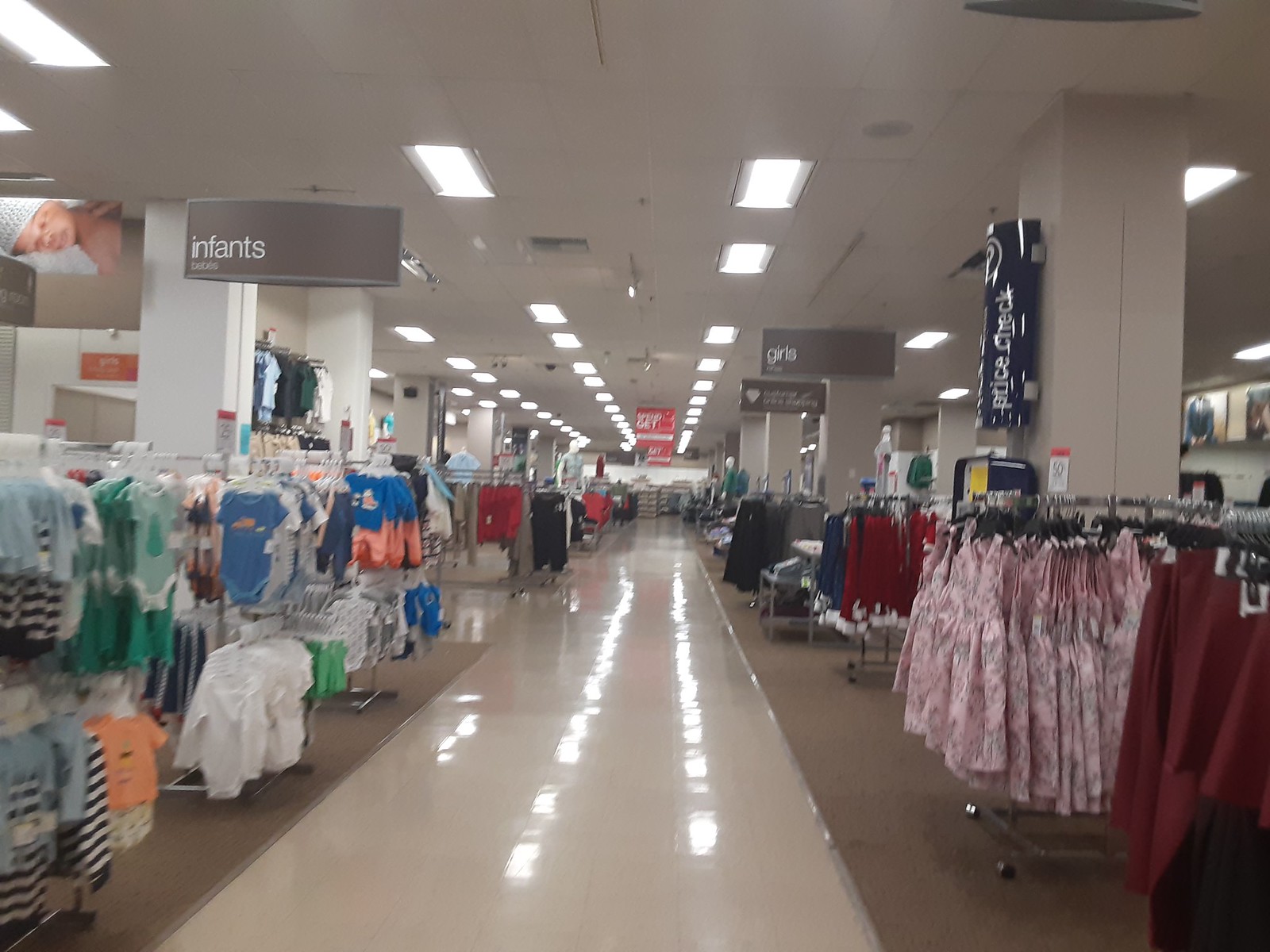The image depicts an aisle in a department store, specifically in the infant and girls clothing sections. The aisle features a long, polished white tiled floor that reflects the recessed fluorescent lighting from the white, grid-style ceiling above. To the left, there's a circular grey sign that says "Infants," accompanied by an image of an infant with a beanie, signaling the start of the infant clothing area. This section showcases a variety of infant clothes hanging on steel racks with white hangers, including blue, green, and white onesies, orange shirts, striped outfits, pajamas with blue tops and orange pants, and an assortment of other brightly colored garments. Additionally, some infant clothes, such as red sweaters, are visible behind the main display.

On the right side of the aisle, a brown sign with white lettering indicates the "Girls" section, where a variety of pink flowery dresses, maroon skirts, and red sweaters are displayed. There are also noticeable racks of red and blue jackets behind the pink dresses. A significant feature on the right side is a blue "Price Check" sign attached to a black round object on a pillar, allowing shoppers to check item prices conveniently.

The aisle extends straight ahead, bordered by various racks of clothing, and is intersected by big square white stone pillars supporting the ceiling. There are glimpses of additional signage further down the aisle, including orange signs, although the text on these is not readable. There's also a small carpeted area on the left within the infants’ section. The detailed layout and diverse clothing options make for a vivid and bustling shopping environment.